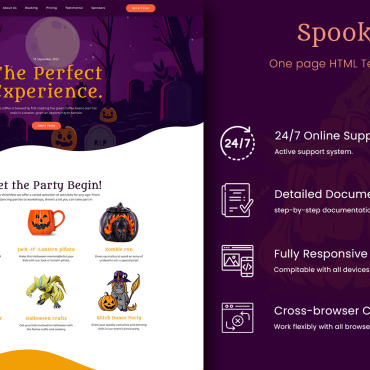This is an image that appears to be a screenshot from a website, formatted as a vertical rectangle. At the top of the image, there are several selectable options, one of which is highlighted in orange, although the text is too small to be legible. Below these options, in orange text, it states "The Perfect Experience."

The background features a spooky graveyard scene with a dark purple sky, a white full moon, tombstones, and several small, glowing orange jack-o'-lanterns. Beneath the highlighted option, an orange button can be seen, accompanied by the text "The Perfect Experience."

Further down, the caption "Let The Party Begin" is displayed, above four distinct images lined up horizontally. The first image is of an orange jack-o'-lantern-styled mug with a black face. The second image shows a little black pumpkin with what appears to be flames on it. In the bottom left quadrant, there's a yellow and green toy. To its right, an illustration of a little witch wearing a hat is positioned next to a jack-o'-lantern.

On the right side of the image, the text "Spook" appears in the top right corner, followed by "One Page HTML" in orange. The background in this section is dark purple. Further down, information about features is provided: "24-7 Online Support," "Detailed Document," "Fully Responsive," and "Cross-Browser." Each feature is paired with white emblems.